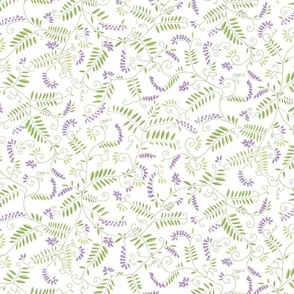This image showcases a detailed, abstract floral pattern primarily composed of green fern-like leaves with long stems and multiple smaller offshoots. Interspersed among these are clusters of lavender and purple flowers, varying in size. The pattern appears irregular and repetitive, giving it a seamless quality akin to a fabric swatch, wallpaper, or wrapping paper. The background of the image is white, enhancing the delicate, fine illustrations of the plants and vegetation. Colors in the design include medium green for the ferns and darker lavender for the flower clusters, creating a visually pleasing contrast against the white canvas. The elements swirl and intertwine, forming a sophisticated, all-over ditzy print with no definitive focal points, adding to its abstract and intricate nature.